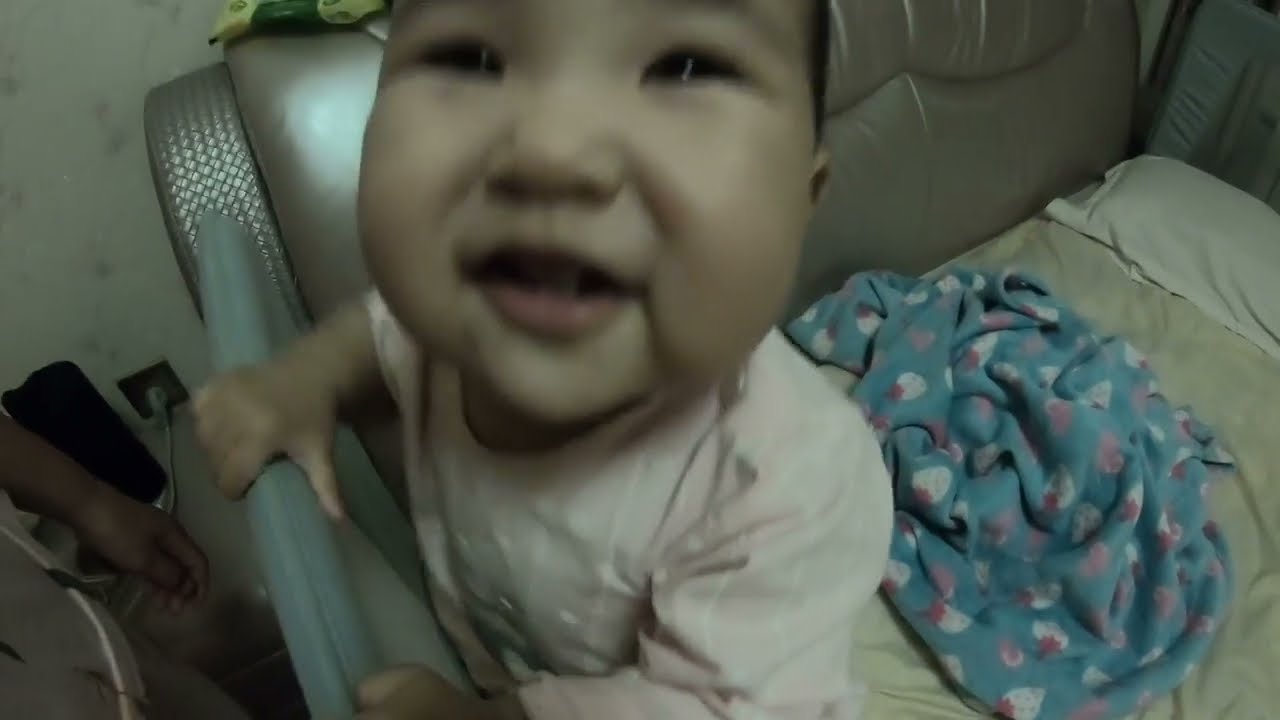In this image, we see a very close-up shot of a smiling infant, likely a little over a year old. The child's face is so close to the camera that it appears somewhat blurred. The baby, possibly a girl given the pink outfit, is standing inside a crib and holding onto its side rail. The crib is cushioned with a light metallic pink and pearl-colored fabric. Behind the child, a blue and pink blanket with some patterns is thrown on a tan mattress sheet, accompanied by a white pillow. The wall behind the crib is mostly white with some gray spots, featuring an outlet with something plugged in. In the background, to the left side of the image, a person's hand wearing a light-colored shirt is visible, extending towards the child. The baby appears happy, with an open mouth, looking joyfully towards the camera.